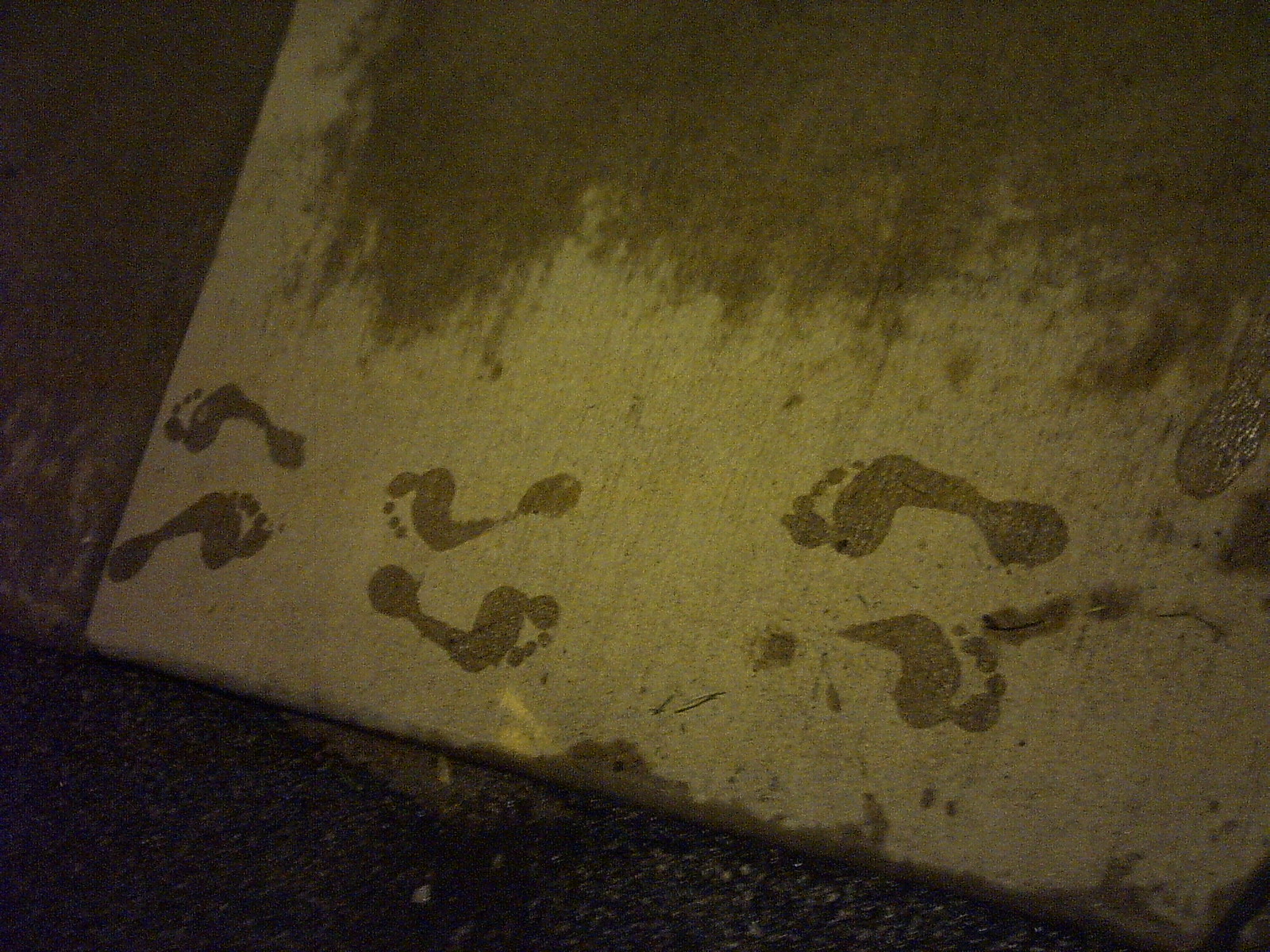The image captures a large concrete slab, possibly a section of a driveway or sidewalk, with a distinct appearance due to varying shades and textures. The lower portion of the slab is a lighter gray, contrasted by a much darker upper portion that appears wet, perhaps from rain or a spill, giving it a mottled look. The edges of the photograph are notably black, adding to the overall dim and moody atmosphere of the image.

In the lower section, what looks like black gravel or rock is visible, adding another layer of texture to the scene. Notably, there are three sets of stenciled or painted footprints on the lighter gray area, indicating that they are not actual human prints due to their narrow shape. These footprints are spaced in a way that suggests someone may have been hopping or moving playfully across the slab, contributing an element of human interaction to the static scene. 

In the upper left-hand corner, the concrete appears darker, almost black, adding depth and contrast to the overall composition. The play of light and dark, along with the scattered footprints, creates a narrative of movement and contrasting elements within this seemingly mundane urban landscape.